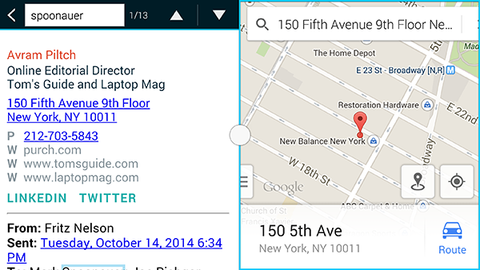The image showcases a split-screen layout with two boxes side-by-side. 

On the right-hand side, there is a Google Maps interface displaying a map with a marked location. The address bar at the top contains "150 5th Avenue 9th Floor, New York, NY." The map features a red marker indicating the New Balance New York location, along with nearby landmarks such as a Restoration Hardware and a Home Depot. At the bottom of the map, the address "150 5th Ave, New York, NY 10011" is listed, along with an icon of a blue car accompanied by a button labeled "Route" that presumably offers navigation from the viewer's current location to the specified address.

On the left-hand side, there is a detailed contact information section. At the top, a white bar displays the name "Avram Pilch," followed by the title "Online Editorial Director, Tom's Guide and Laptop Magazine" beneath it. The address is listed again as "150 5th Avenue 9th Floor, New York, NY," alongside a phone number and multiple website links. Underneath this information, there are LinkedIn and Twitter icons for social media connections. At the bottom of this section, a note reads "From Fritz Nelson, sent Tuesday, October 14th, 2014, 6:34 PM," highlighted in blue.